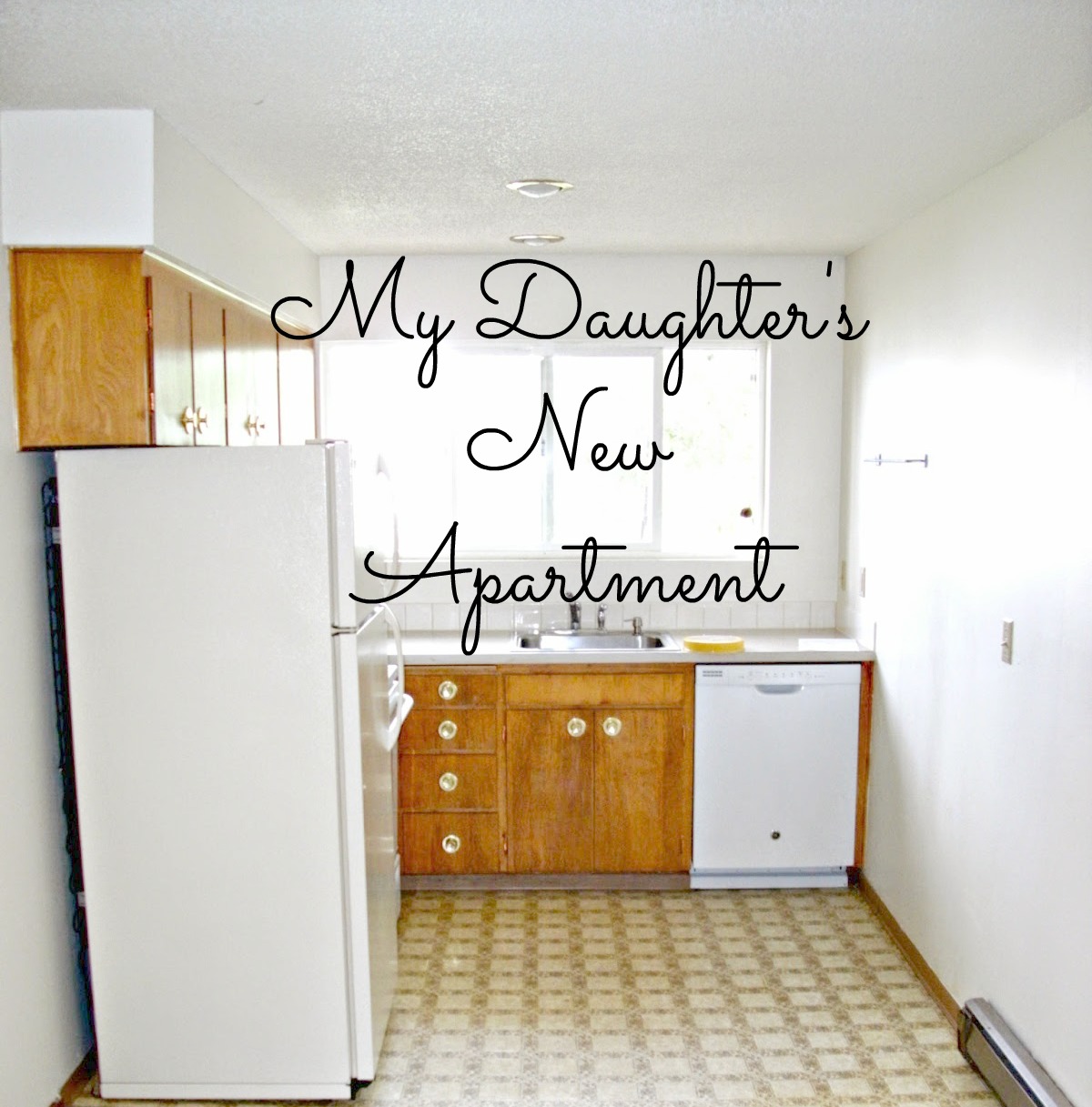The photo shows a small, basic kitchen, typical of an apartment. The kitchen is framed by two side walls and a back wall, all painted white, with a window on the back wall that has a large sliding section flanked by two additional panels, flooding the space with natural light. Beneath this window is a double sink with a cupboard underneath and flanked by four drawers. To the right of the sink, the countertop turns into an L-shape. 

Above the countertops and appliances on the back wall, there are three sets of wooden cabinets. Along the right side beneath the counter is a white dishwasher, while the far left side features a white refrigerator with a top freezer, fitting snugly under the overhead cabinets. The floor is covered with beige and green linoleum. Across the photo, in black cursive text, there is a caption that reads, "This is my daughter's new apartment."